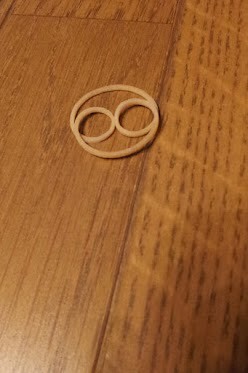A detailed color photograph, displayed in portrait style, captures a light brown wooden table with distinctive darker striations tilted diagonally to the right. The wooden surface, polished to a shine suggesting overhead lighting, features a single rubber band intricately twisted and laid at the center top. The rubber band forms a larger circular shape with two smaller intersecting circles inside, resembling a human face. This composition rests atop a slat or small divider present on the table, adding an element of depth and separation. The rubber band itself is a pale beige-brown color.